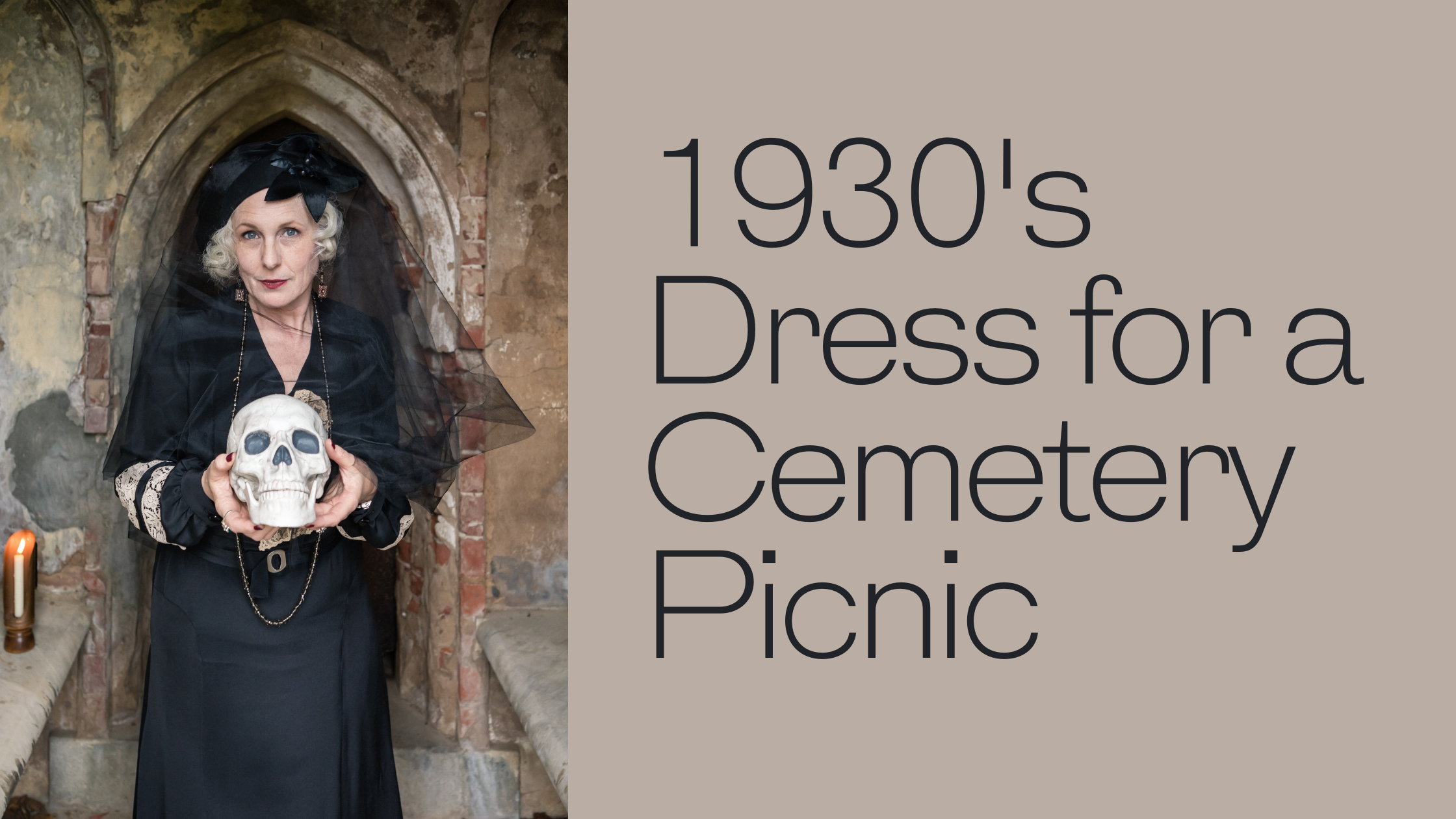In this captivating rectangular image, an older woman with gray hair is centrally featured, dressed in a striking black dress adorned with intricate brown designs. She stands poised in what appears to be a stone archway or hallway, with benches flanking her on both sides—one of which holds a lit candle. The setting conveys a somber, antiquated atmosphere. Her black fancy hat, embellished with a bow, sits elegantly atop her head. The woman’s dark eye makeup and dark brown earrings add to her gothic appearance. In her hands, she holds a skull, and around her neck hangs a long, dark necklace that extends below the skull. She gazes directly into the camera with a piercing, almost haunting look. The image is divided, with the left side featuring the photograph of the woman and the right side bearing a tan section that reads, "1930s Dress for a Cemetery Picnic," encapsulating her attire and the eerie scene she embodies.